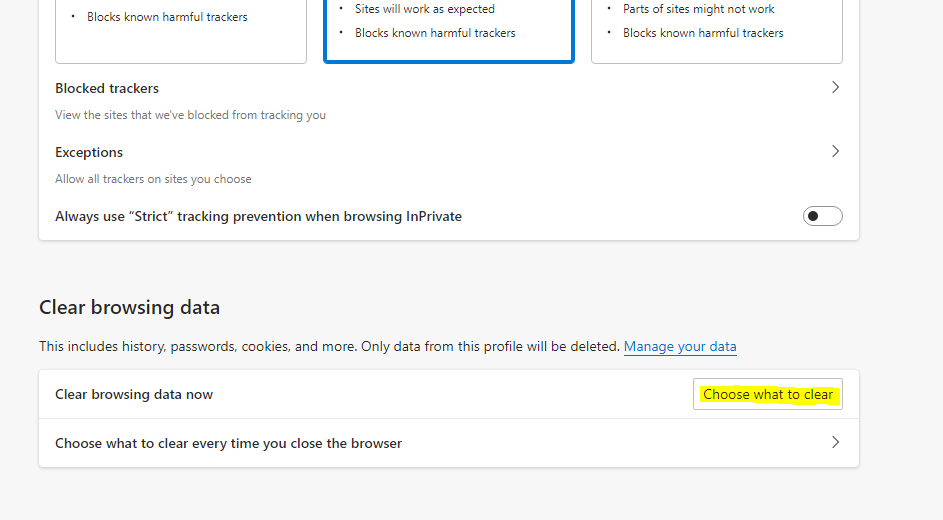**Descriptive Caption:**

This webpage falls under the category of website settings and focuses on privacy and tracking prevention. The page appears partially cut off, revealing three main sections at the top, each distinguished by different privacy levels and their potential impact on website functionality. The section on the left, labeled "Blocks known harmful trackers," signifies a stringent setting where harmful trackers are blocked. The middle section, highlighted with a blue outline, states "Sites will work as expected" while still blocking known harmful trackers, indicating a balanced approach that maintains site usability. The third section on the right indicates that "Parts of sites might not work" due to the blocking of harmful trackers, suggesting a more aggressive blocking mode.

Below these categories, additional privacy-related options are available: "Blocked trackers" provides a view of the sites that have been prevented from tracking the user. The "Exceptions" section offers the ability to allow trackers for specific sites chosen by the user. A setting titled "Always use strict tracking prevention when browsing in private" is present, advocating for higher privacy standards during private browsing sessions.

Further down, options for managing browsing data are listed. "Clear browsing data" includes a link to actions like deleting history, passwords, and cookies, with a note that only data from the current profile will be erased. The link to execute this action is labeled "Clear browsing data now." Additional choices are provided for clearing data, including "Choose what to clear" and the option "Choose what to clear every time you close your browser."

This page is a comprehensive interface for managing privacy and data handling, emphasizing user control over tracking and data retention.